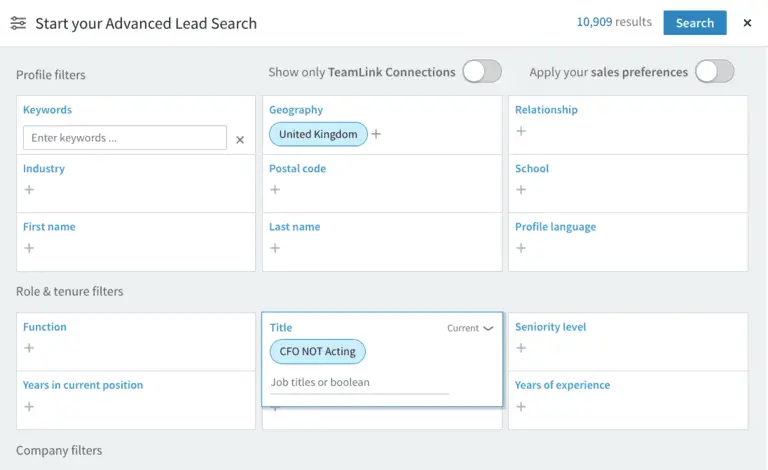The image showcases an advanced lead search interface with a predominantly gray background and sections with white backgrounds. In the top-left corner, a screen displays the prompt "Start your advanced lead search." To its immediate right, the interface shows a result count of "10,909" with a blue search button and an 'X' for closing.

The screen is divided into several sections:

1. **Profile Filters** (Top Section):
    - **Keywords:** Contains an input field labeled "Enter keywords" in blue writing.
    - **Industry:** A dropdown or field to specify the industry.
    - **First Name:** An input field for entering the first name.
    - **Geography:** Options available are "London" or "United Kingdom."
    - **Postal Code:** An input field for the postal code.
    - **Last Name:** An input field for entering the last name.
    - **Relationship:**
      - **School:** A field for specifying the school.
      - **Profile Language:** A dropdown or field for selecting the profile language.
    - Above these filters are two toggle options:
      - **Show only team connections:** Currently toggled off.
      - **Apply your sales preferences:** Currently toggled off.

2. **Role and Tenure Filters** (Middle Section):
    - **Function:** A dropdown or field to specify the function.
    - **Years in Current Position:** An input field or range selector.
    - **Title:** Set to "CFO" within a blue oval shape, indicating the title filter is applied.
    - **Job Titles or Boolean:** An input field for job titles or Boolean search terms.
    - **Current:** Displayed at the top right of this section.
    - **Seniority Level:** A dropdown or selector for seniority level.
    - **Years of Experience:** An input field or range selector.

3. **Company Filters** (Bottom Section):
    - A partial view of this section indicates there are additional company-specific filters below.

The UI elements are well-organized to facilitate advanced searches with specific criteria, enhancing the efficiency of lead generation activities.